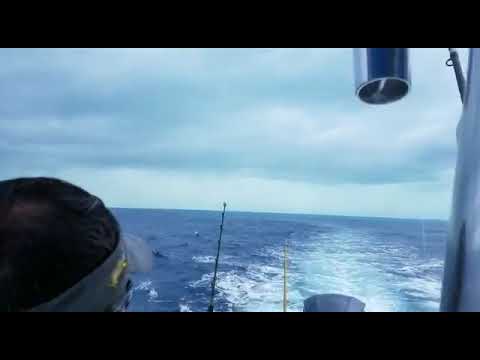The image captures a serene ocean scene from the vantage point of a boat, likely a fishing vessel, evidenced by the two fishing rods visible in the lower portion of the image. The horizon meets the partly cloudy, bright sky about halfway up the image, dividing the blue of the ocean from the light sky. In the bottom right corner, a broad, white water wake is seen, illustrating the boat's motion. On the left side, there's the head of a person wearing a visor, partially obscuring their balding dark hair, while their face remains unseen. A dark-colored object with a gray strip and blurry yellow text, possibly a part of the boat, is seen adjacent to the fishing rods. Additionally, a metal pole extends vertically along the far right edge of the image, and a cylindrical object, likely part of the boat's structure, is situated in the upper right corner, contributing to the composition of the scene. The entire image is framed by a subtle black border at the top and bottom, encapsulating the tranquil yet dynamic maritime snapshot.